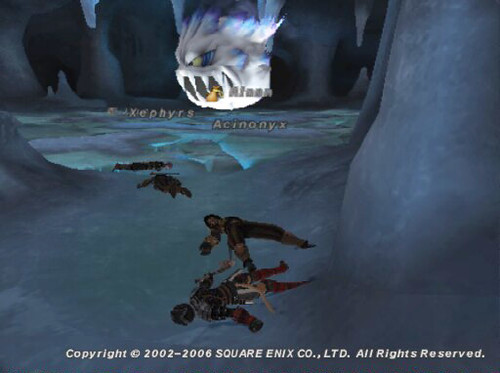The image appears to be a scene from a video game, likely showcasing a dramatic or action-filled moment. The background is predominantly blue, resembling water or a similar fluid environment. In the center, there is a glowing light that draws the viewer's attention. Four human figures are depicted falling amidst this scene; two are smaller and located in the middle, while the other two are more prominent in the foreground. These individuals are wearing costumes or uniforms, hinting at a specific role or character they are portraying. One of them is holding an item that resembles a stick or sword, suggesting they are equipped for combat or adventure. 

Dominating the top portion of the image is a vividly lit, menacing white creature with sharp fangs and a bulging eye. The creature's head features sharp, illuminated spikes, and it has something beige clutched in its mouth. Positioned across this creature is text that reads "A-T-M-A-N" in grey, though the exact wording is somewhat unclear. The background also includes what looks like a cave, adding to the mysterious and adventurous atmosphere of the image. At the bottom, a disclaimer reads: "Copyright 2002-2006, Square Enix Company, Ltd. All Rights Reserved," indicating the game's origin and licensing information.